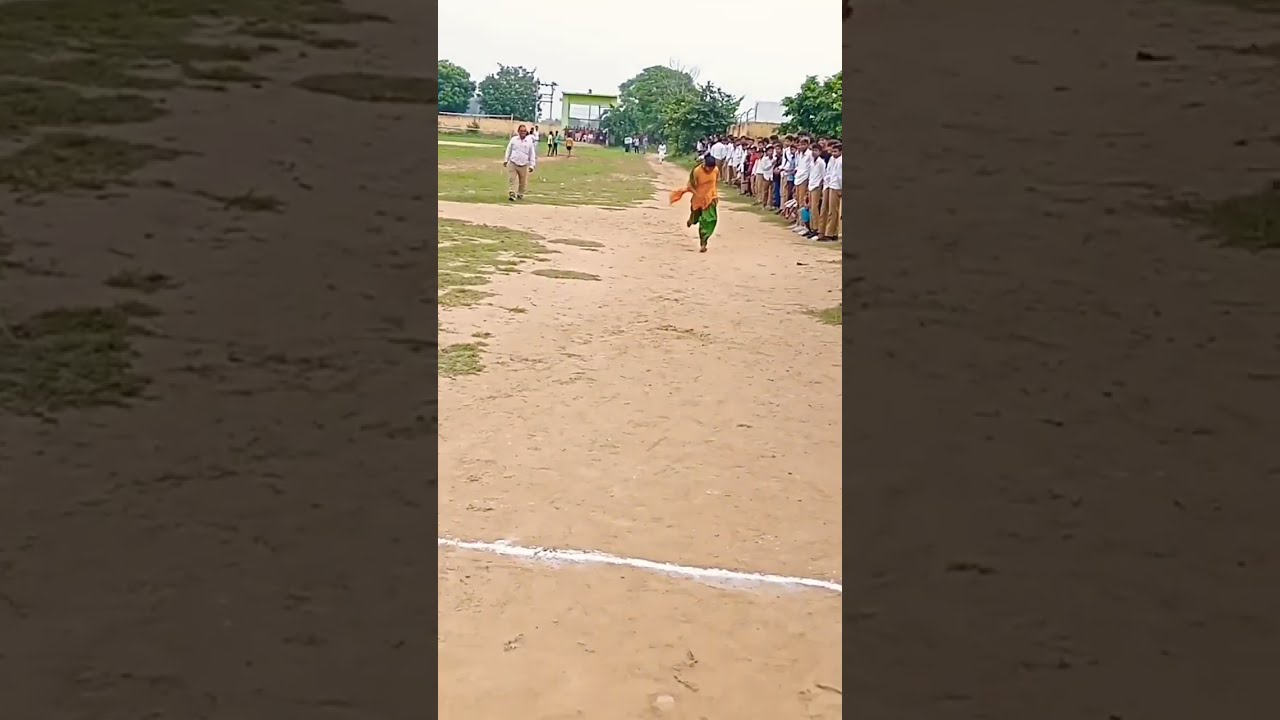The outdoor scene captures a lively moment on a sports field. On the right side of the image, a group of young boys, all dressed in matching white dress shirts and khaki or brown dress pants, stand in a line. These boys, who appear to be students, are watching attentively as a woman in an orange shirt and green trousers runs towards a white chalk line on the ground, resembling a finish line. The field is a mix of sandy and grassy patches, giving a dry, earthy feel to the scene, complemented by earth tone colors like sandy brown, green, orange, and blue. In the background, the field is enclosed by a cement fence, and there's an archway visible on the upper left side, hinting at an entrance to the area. On the left side of the image, an older man, also in a white shirt and brown trousers, walks on the grassy segment. Additionally, there's a badminton or racket net placed on the left side. Dotted throughout the scene are random passersby, including a black woman in an orange shirt and green pants, amidst trees and a partly visible building, indicating a busy, engaging environment typical of a school event.